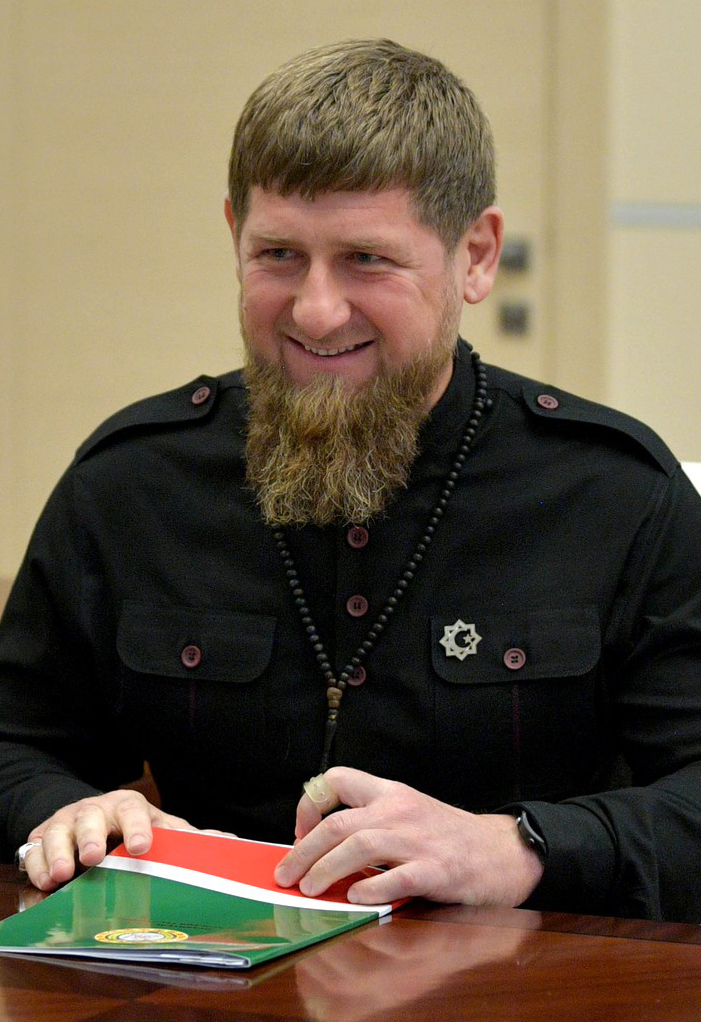A man with short hair and a bushy beard is slightly smiling while gazing upwards to the left, away from the camera. He is wearing a black shirt with buttons down the center and a badge indicative of his religious affiliation is pinned to the buttoned chest pocket. His right hand, adorned with a watch and a possible bandage on one of his fingers, rests on a colorful pamphlet featuring green and orange hues with a yellow circular symbol at the top. His left hand is also placed on the pamphlet, revealing a ring on one of his fingers. Additionally, the man is wearing a necklace that subtly complements his attire and accessories.